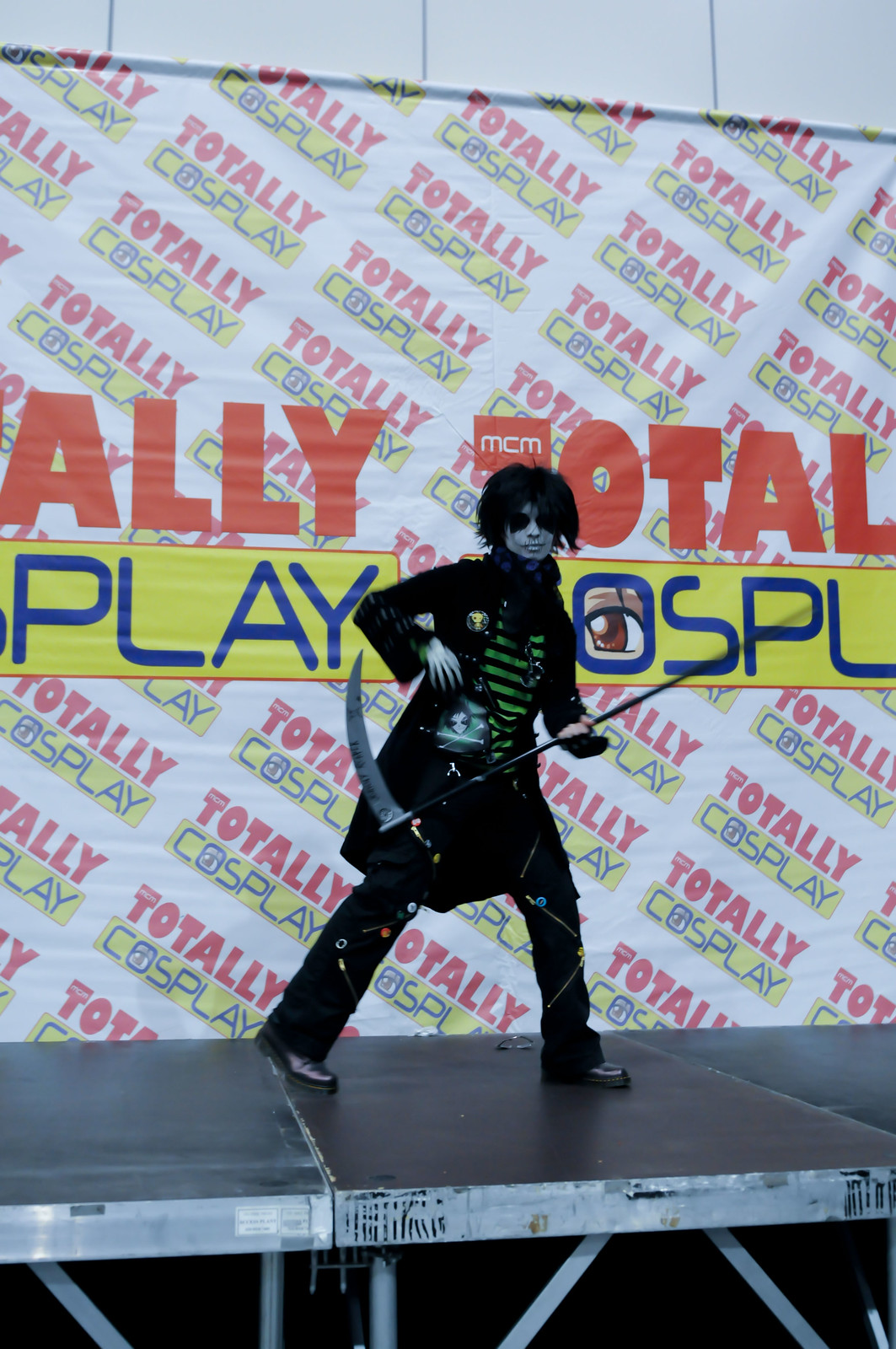The image captures a striking scene at a cosplay event, where a lone figure stands on a small, thin stage supported by metal bars and featuring a brown floor. The backdrop is notably dominated by a large, diagonally-written poster that repeatedly spells out "Totally Cosplay" in a bold red font for "Totally" and framed in a yellow box with blue letters for "Cosplay," some of which are partially obscured. Decoratively, the "O" in "Cosplay" incorporates an image of an eyeball. 

The person on stage is donned in an elaborate costume resembling a Grim Reaper or skeleton character. They wear a long, black coat adorned with zippers and green stripes that mimic ribs on the front, matched with long black pants and black boots. Their face is painted white to simulate a skull, with black circles around their eyes, giving a ghoulish appearance. They complete the eerie look with black shoulder-length hair. In their hands, they brandish a plastic scythe, held upside down as if they are playing it like a guitar. The ensemble also includes various pins and images of anime characters, adding intricate details to the costume.